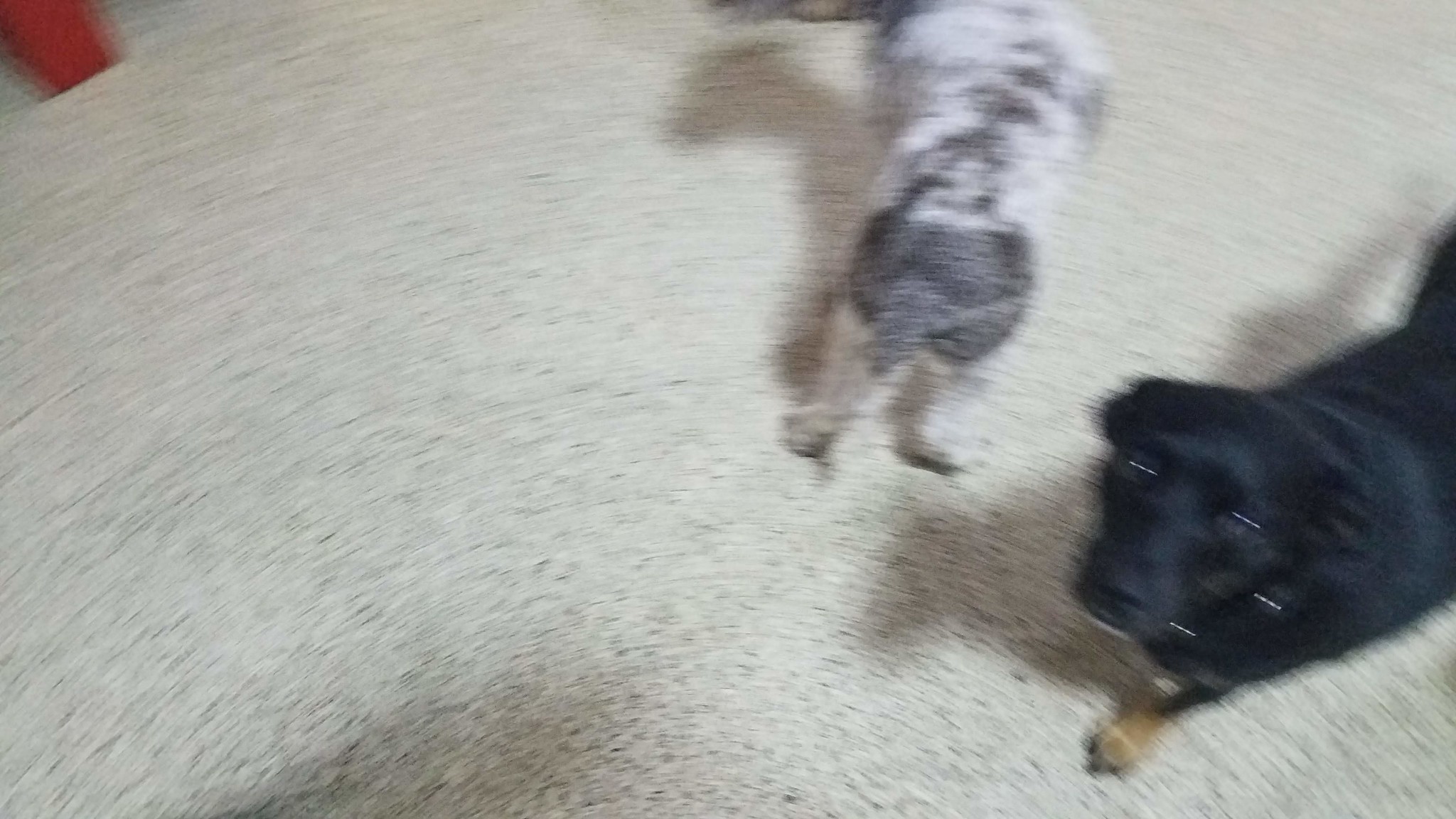This photograph captures a moment in motion, resulting in a very fuzzy and out-of-focus image. The light-colored floor, speckled with black, serves as the backdrop. To the right, a medium-sized black dog with distinct tan paws gazes up at the camera. Adjacent to it on the left is another dog, seen from behind, displaying a striking white and gray brindle coat. The blur and lack of sharpness in the image suggest it was taken while the subjects were moving.